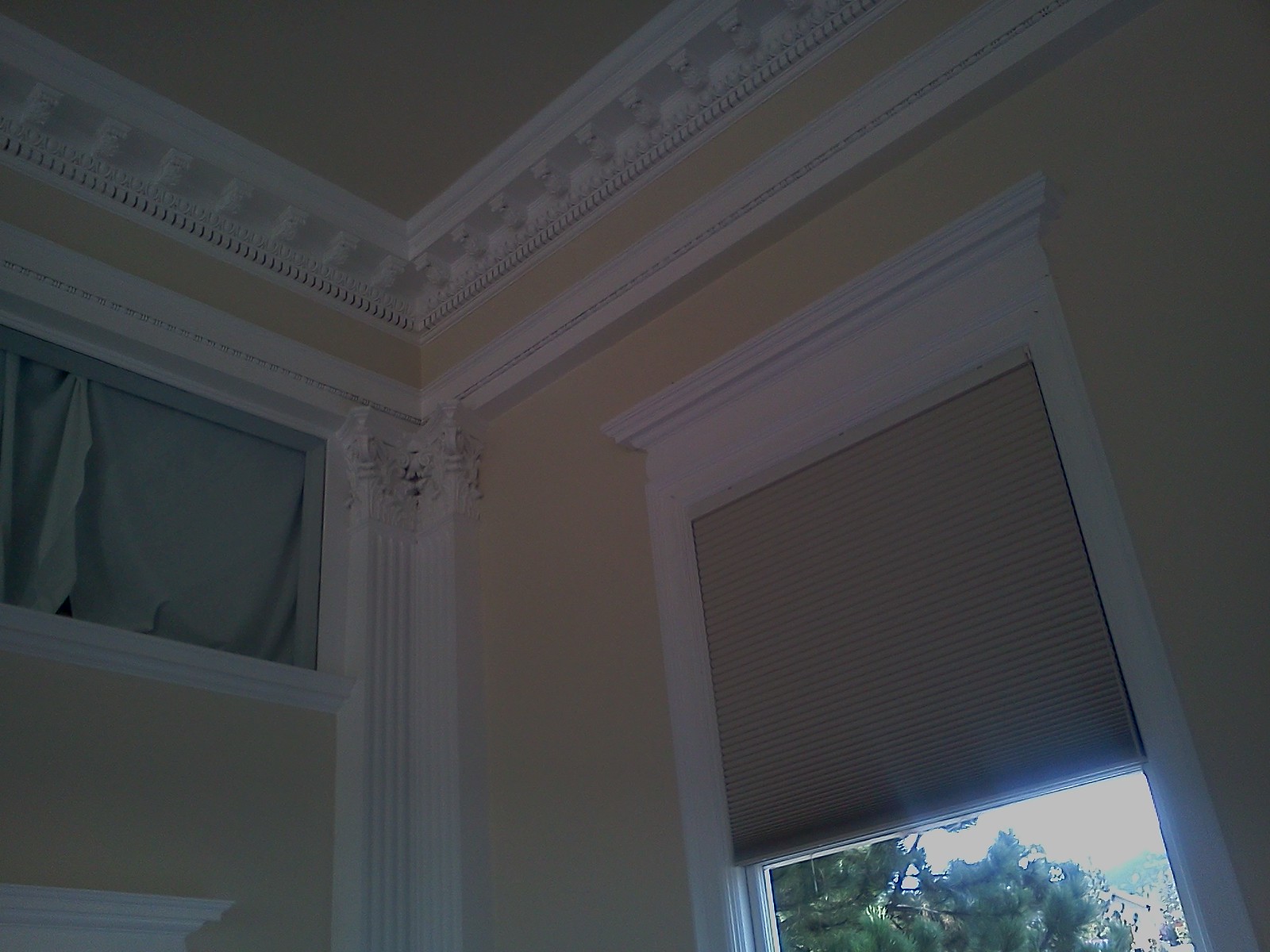This photograph captures the corner of a room with vintage charm, characterized by its ornate crown molding and detailed carvings. The walls are painted in a pale yellow or cream shade, adding a warm ambiance to the space. On the right, a large window features cream-colored brown blinds drawn halfway up, revealing a lush evergreen tree outside against a backdrop of a bright blue sky, accentuated by deep white from strong sunlight. The window frame is lined with white wood, with additional grouting visible above and around it. To the left, a smaller window is partly covered by a curtain, its bluish or greenish hue softened by low lighting. The ceiling is yellow, bordered with the same elaborate white molding that follows the lines of the walls and windows.